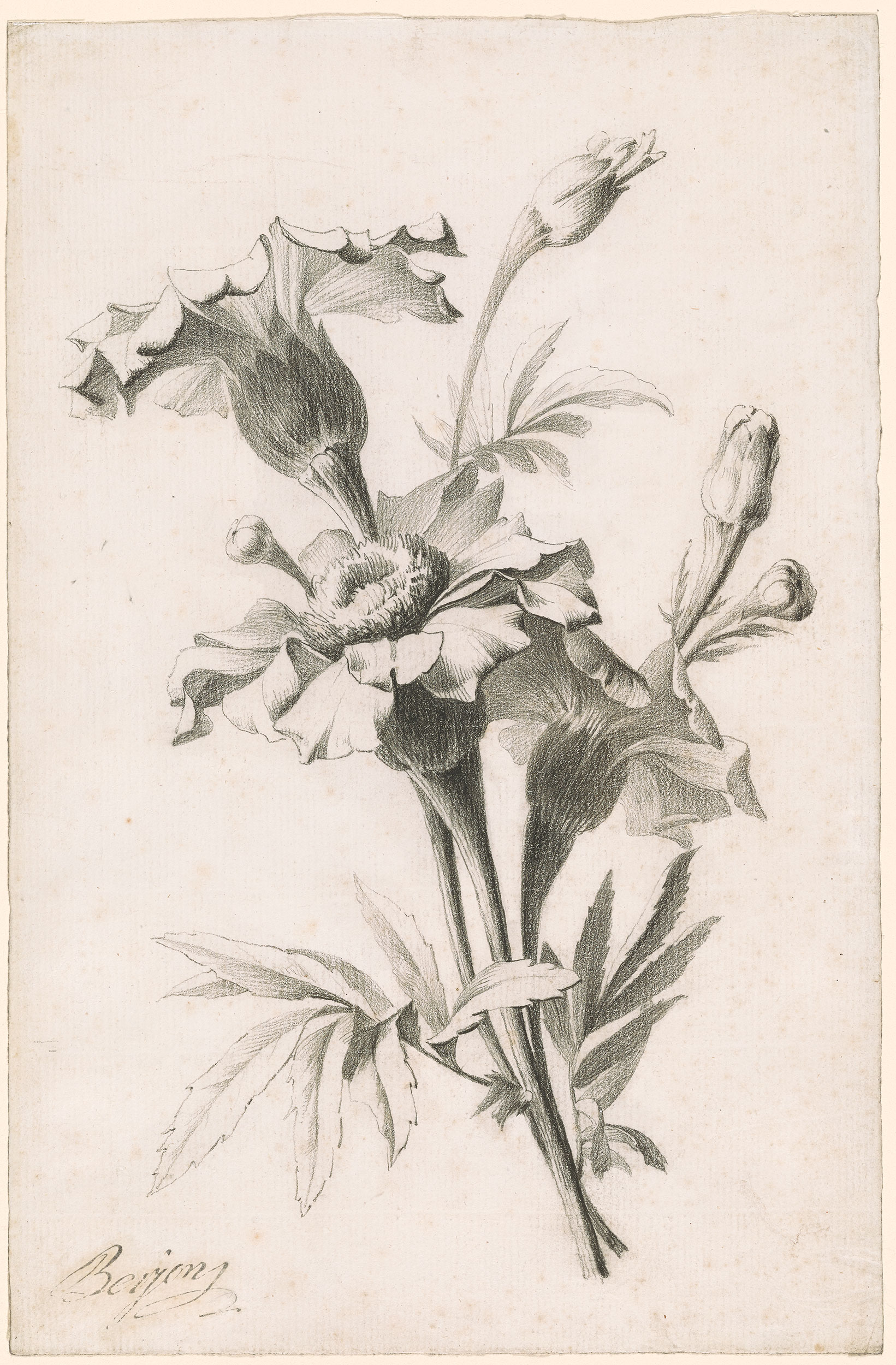This detailed pencil sketch in portrait mode features a botanical illustration of a plant, resembling a thistle or marigold, set against a cream-colored, slightly yellowed background. The aged appearance suggests it's from an old book or card. The artistic rendering is in black and white, with some accents in green. The plant has two main stems rising from the bottom right center, each bearing multiple black stalks that give rise to large, wrinkled petals surrounding a protruding center circle. Additional offshoots with smaller buds and detailed, long serrated leaves extend from the main stems. The artist's signature, an elegantly scripted and somewhat ambiguous "B-E-I-J-O-N-G-J" or "B-E-R-I-O-N-S" with a flourish, is located in the bottom left corner of the page.